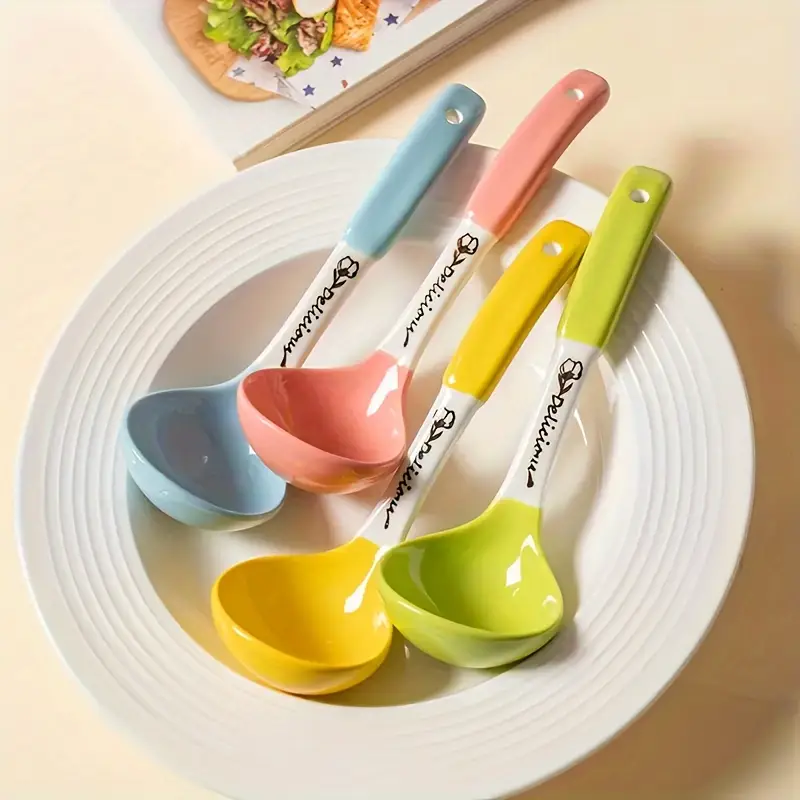A vibrant and colorful assortment of four serving spoons is artistically arranged in a shallow, white ceramic bowl with etched concentric rings along its rim. The spoons, designed in a modern style, feature pastel colors of light blue, pink, yellow, and lime green. Each spoon has a unique handle that transitions halfway from its respective color to a white section inscribed with the word "delicious" in a special font, accompanied by a delicate flower motif. The ceramic bowl rests on a cream-colored tabletop, casting subtle shadows. Positioned behind the bowl is a gray book or menu, displaying a photograph of food on a wooden tray adorned with leafy greens and what appears to be a piece of cooked meat, enriching the overall warm and decorative ambiance.